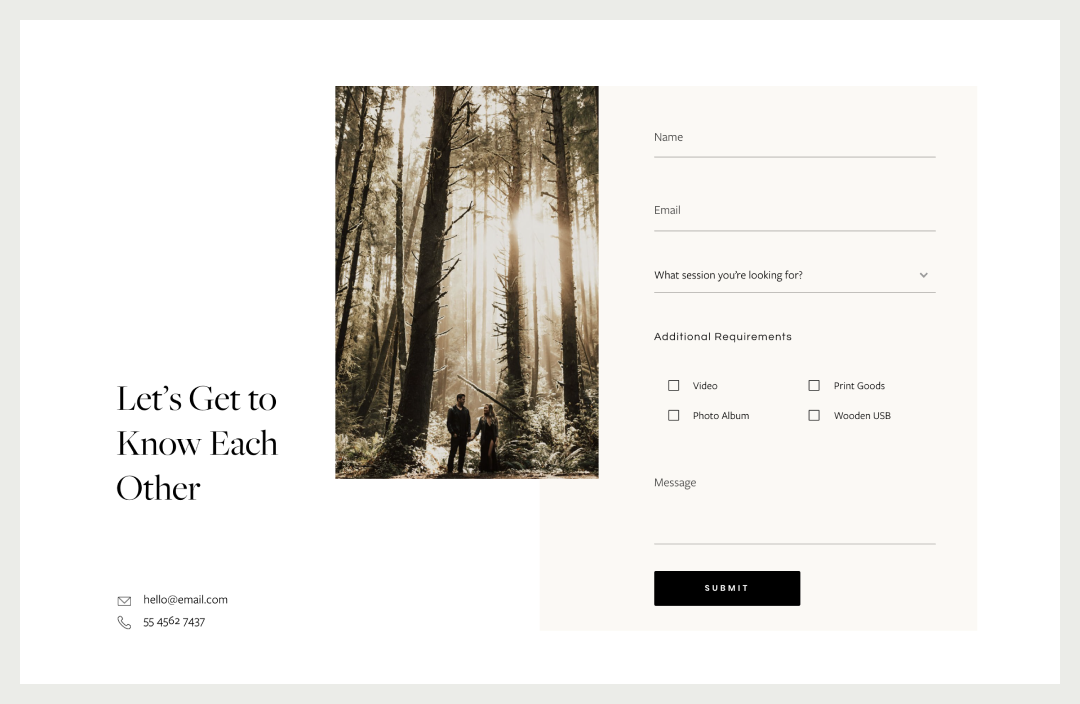The image is a rectangular design, oriented horizontally, with a proportional length greater than its height. It features a moderately thick gray border and a white background. On the left side, towards the lower portion, bold text reads "Let's get to know each other" in the largest font size on the image. Immediately below this text, there is a contact email indicated by an envelope icon, stating "hello at email.com," followed by a phone icon and the number "554-562-7437."

Central to the design is a sepia-toned photograph showcasing a majestic forest of towering pine trees. At the bottom of this forest scene, a man and a woman are depicted holding hands and gazing at each other, appearing diminutive against the backdrop of the trees.

To the right of this image, the following elements are methodically arranged: 

1. A section labeled "Name" followed by a blank line.
2. A section labeled "Email" followed by a blank line.
3. A dropdown menu labeled, "What session are you looking for?"
4. A section labeled "Additional requirements" with checkboxes for options including: "Video," "Photo Album," "Print Goods," and "Wooden USB."
5. A section labeled "Message" with an accompanying blank line.
6. A "Submit" button prominently placed for users to finalize their inputs.

The overall palette consists of subtle grays, white, black, sepia tones suggesting brownish hues, minor touches of green, and hints of blue, creating a visually engaging and harmonious design.